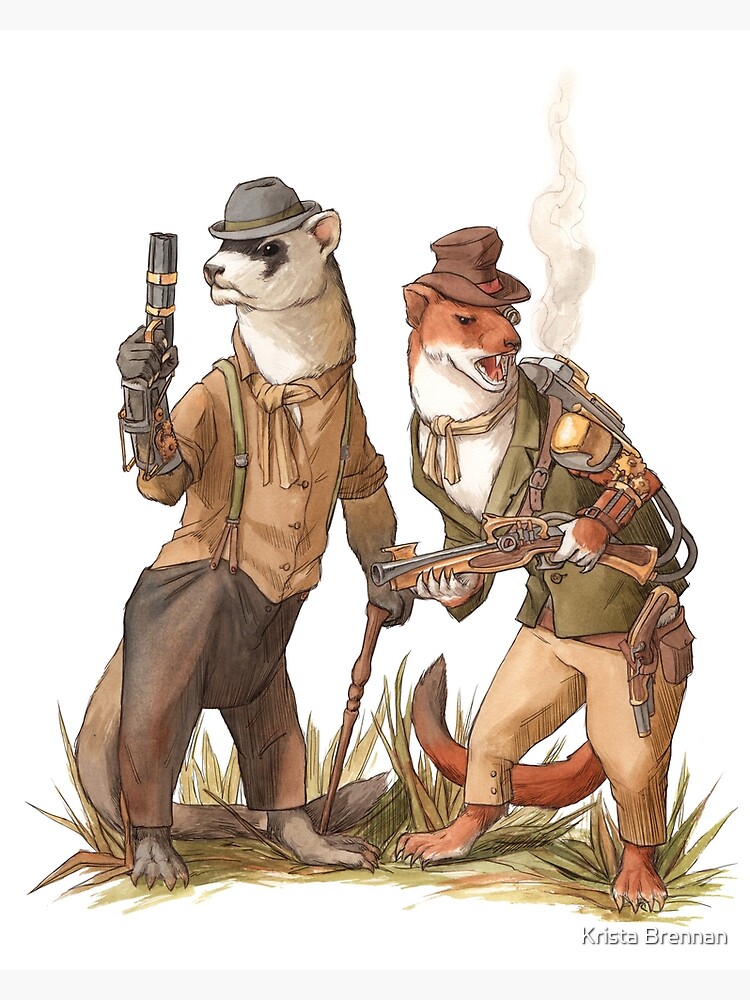This detailed illustration depicts two anthropomorphic ferrets dressed in military-like steampunk attire, amidst a grassy field with a white background and hints of smoke on the right. The ferret on the left, resembling a meerkat with a white and black coat, sports a gray top hat, an orange shirt under brown overalls, and black pants. This ferret holds a pistol in one hand and a cane in the other, with a scarf tied around its neck and a noticeable long tail. The ferret on the right, with an orange and white coat, dons a brown hat, a green dress coat, and khaki pants. It is armed with a rifle and another firearm at its hip, and it carries a steampunk-styled backpack featuring shoulder armor. Both ferrets have expressions indicating alertness, with the left one looking to the left and the right one to the right with an open mouth. The scene is set against a greenish-yellow grassy field, adding a whimsical yet adventurous feel to the overall composition, signed by Krista Brennan.